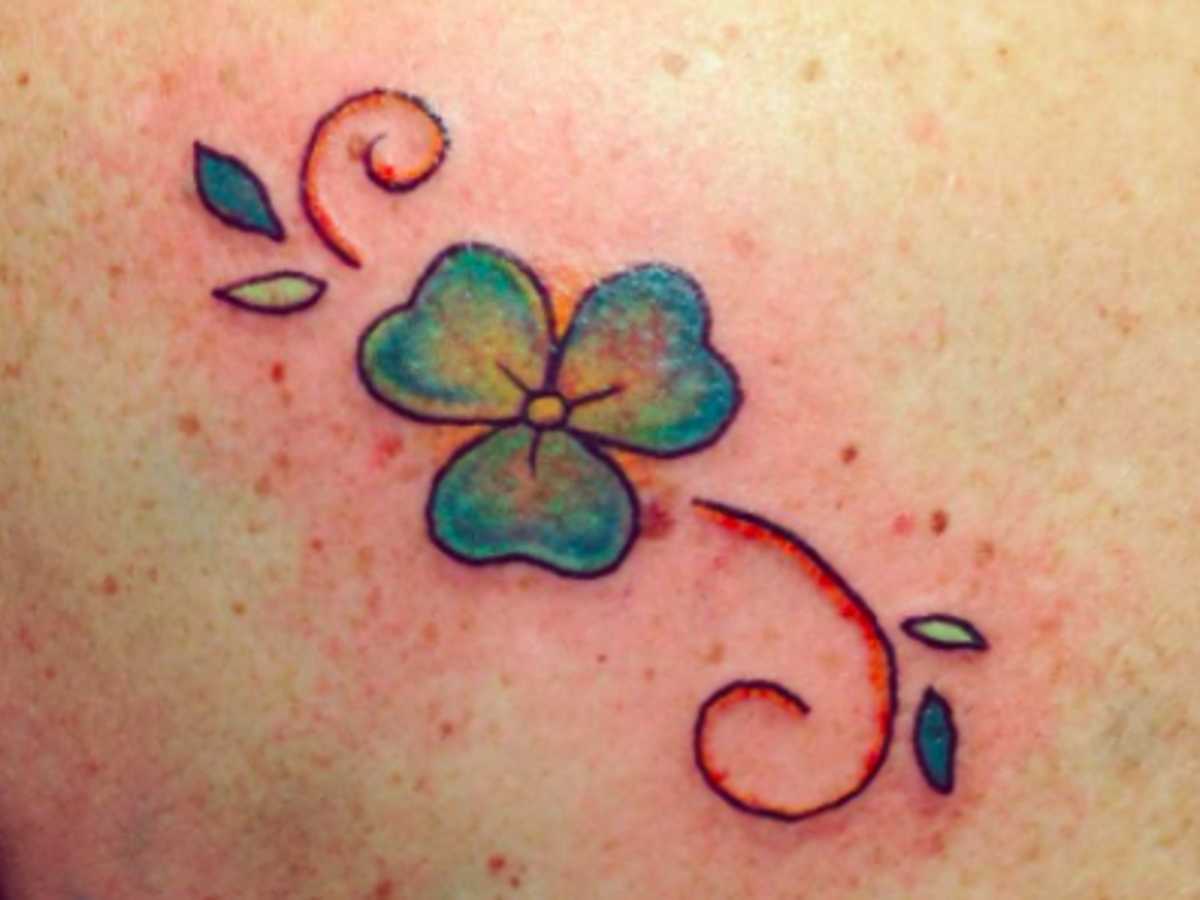This up-close photograph showcases a freshly completed tattoo on white, freckled skin. The skin around the tattoo is noticeably red and inflamed, indicating it was just finished. The centerpiece of the tattoo is a green three-leaf clover, adorned with a yellow circle in the middle, which adds a floral touch to the design. Flanking the clover are intricate black and red filigree swirls that curl outward in opposite directions. Enhancing the symmetry are two decorative leaves, one light green and the other dark green, mirror-imaged on either side of the central motif. The careful detailing and vibrant colors make this new piece of body art particularly striking against the reddened, freckled canvas.